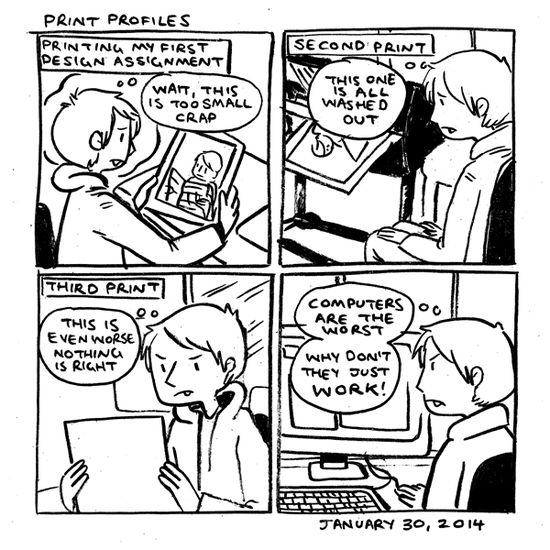This is a black and white comic titled "Print Profiles," consisting of four panels. The first panel features a frustrated boy holding a picture with the caption, "Printing my first design assignment. Wait, this is too small! Crap!" In the second panel, the same boy is sitting on a chair, looking at a new print and saying, "Second print: This one is all washed out." The third panel shows him even more exasperated, holding a sheet of paper and exclaiming, "Third print: This is even worse. Nothing is right." In the fourth panel, the boy is angrily working at a computer, thinking, "Computers are the worst. Why don't they just work?" At the bottom right of the comic, the date "January 30, 2014" is displayed.